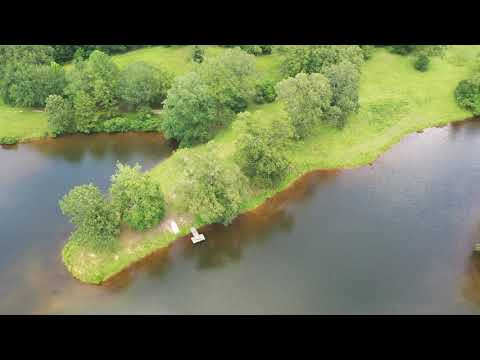This aerial photograph captures a high-angle view of a lake surrounded by verdant, grassy, and hilly land. The landscape slopes gently towards the clear, sediment-tinged water, which appears light tan in color. Scattered around the area are low-lying, bushy trees, roughly 20 feet tall. A notable feature of the scene is a small peninsula, extending diagonally from the top right to the bottom left of the image, covered in grass and trees. At the tip of this mini peninsula, there is a small dock or pier, possibly used for mooring a canoe, giving the impression of a remote, off-the-beaten-path location, potentially within a national park. The water also appears to fork into two distinct areas, creating a cove-like separation.